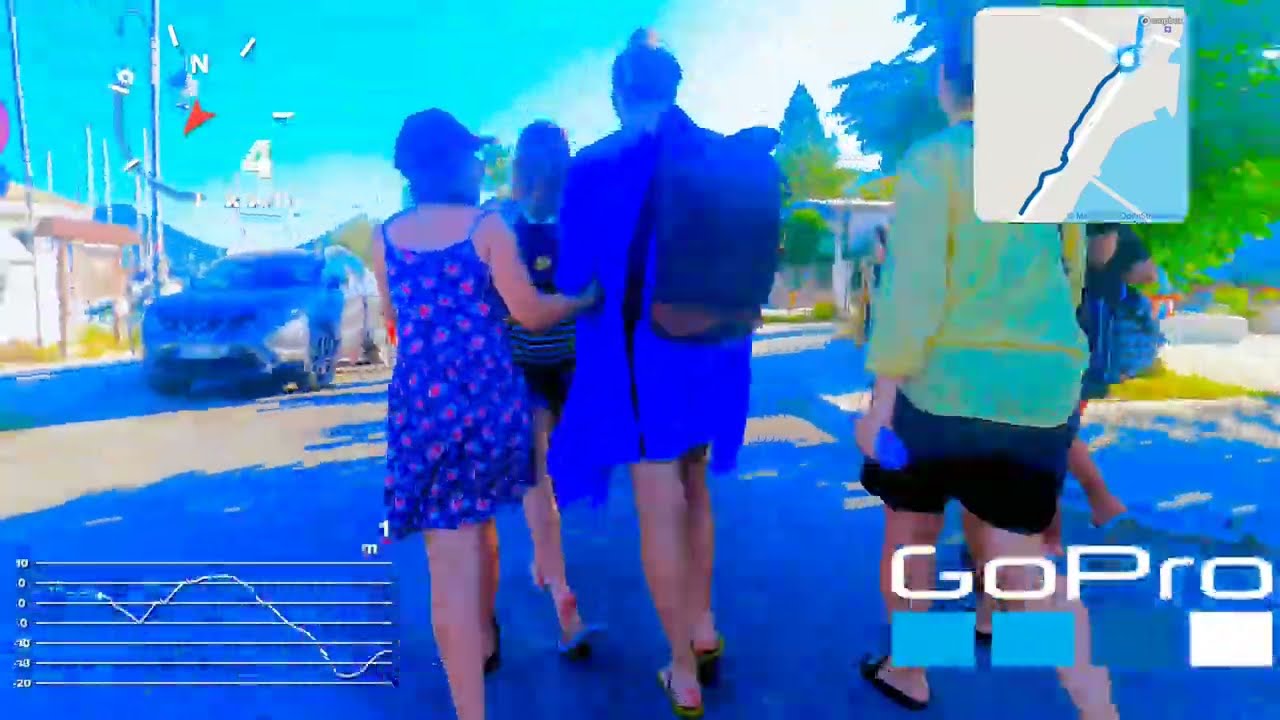This photograph, approximately six inches wide by three inches tall, depicts a group of people walking on a road in an outdoor setting during the daytime. The image has a blue color filter applied, giving it a slightly pixelated appearance. The group, consisting of at least three women and one man of Caucasian descent, walk away from the camera with their backs facing us. Vehicles can be seen passing by on the left side of the road.

Several digital elements are overlaid on the photograph. In the upper left corner, a compass icon is visible, showing north at the top and a red arrow pointing towards the 8 o'clock position. The upper right corner features an overlaid map icon indicating the group's route from the lower left to the upper right corner of the photograph.

In the lower left corner, there's a bar graph with seven horizontal bars marked with values starting from ten, descending to zero, and dropping into negative values. Also in this corner, the graph's line starts around zero, dips, rises, and then plunges into the negative range. The lower right corner displays the text "GoPro" in bold white print. Below this text, there are four small squares: two light blue, one dark blue, and one white.

The background includes a blue sky in the upper left and green trees in the upper right, contributing to the overall outdoor ambiance of the scene.